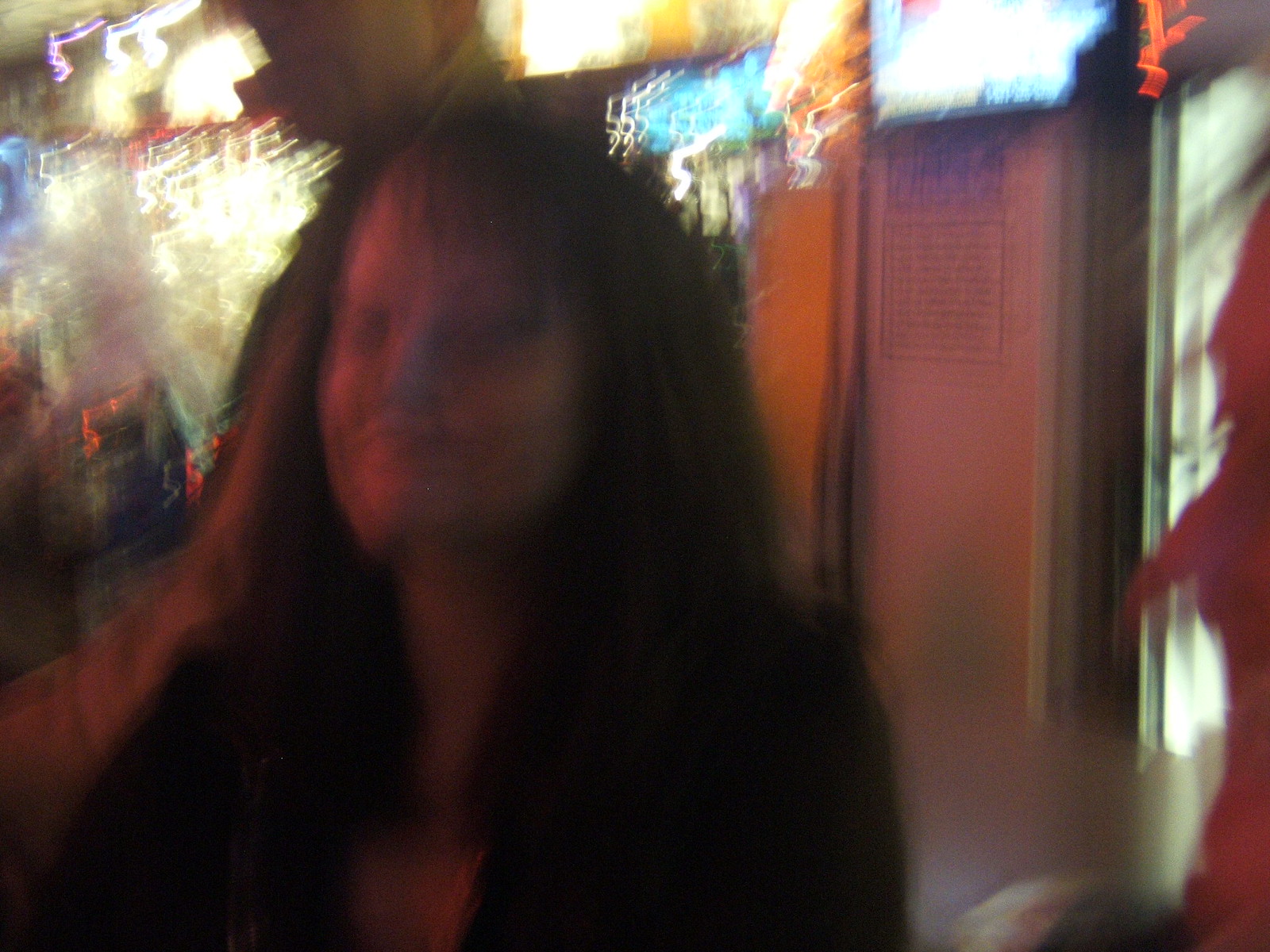The image is a super blurry photo featuring a woman at the center with bangs and long brown hair that extends a bit past her shoulders and blends into her dark shirt, possibly black. Her facial features are indistinct, especially her eyes and lips. The background is vibrant and colorful, suggestive of a lively setting like a bar, restaurant, or club. Bright white and blue lights can be seen behind her, with additional orange and red lights that resemble Christmas decorations. There's also a bright glare in the upper right corner which seems to come from a television or a sign. On the right side, there’s a faint outline resembling a partially visible face in profile, evoking the character Snow Miser from the Christmas cartoon. The overall scene is bustling with blurred signs that hint at a dynamic and festive atmosphere.